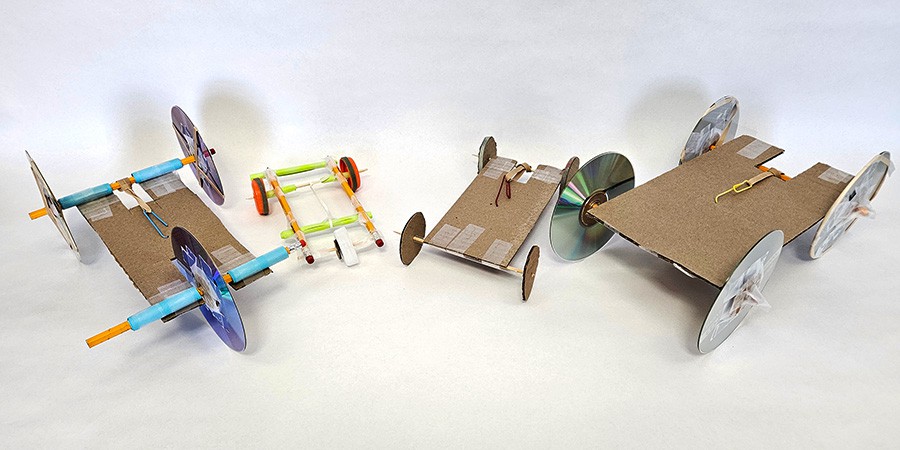In this horizontal image set against a light beige background, four handcrafted cardboard carts of varying sizes and colors are aligned side by side. The carts, resembling miniature wagons, are constructed from flat cardboard bases with CD discs for wheels, held together by toothpicks and pencils acting as axles. The CD wheels display a range of colors including gray, purple, and green, and cast minor shadows on the white backdrop, suggesting an artificial light source. This intricate arrangement, possibly the result of a middle school science project, showcases an elementary exploration of physics concepts such as velocity and gravity, reflected in the careful assembly and varied design of each cart.